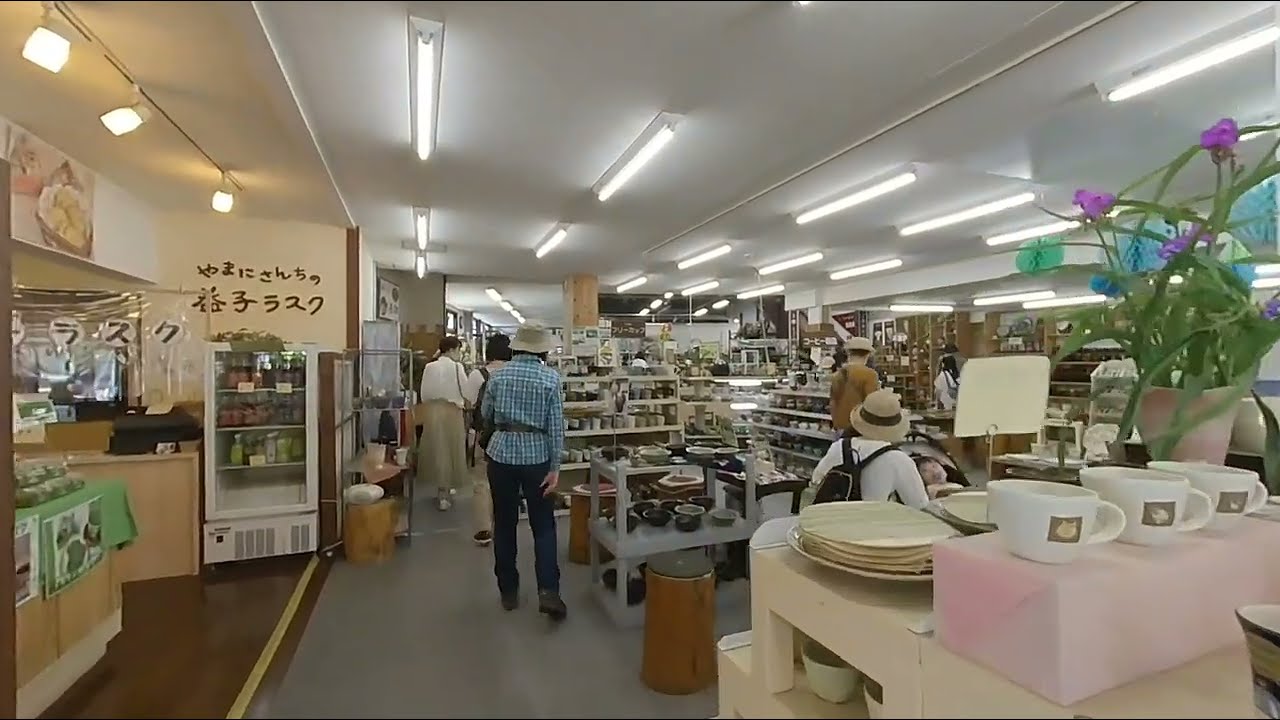The photograph captures the bustling interior of a Japanese department store, reminiscent of Williams and Sonoma or Pottery Barn but distinctly Asian with Japanese lettering adorning the walls. The spacious store features a harmonious blend of white shelves and beige countertops, illuminated by long fluorescent tube lighting on a white ceiling. The floor transitions from brown with a yellow stripe on the left side, hinting at an eatery or bakery area complete with a small white cooler and beige counter, to a grey tile in the main shopping area.

Scattered across the store, about ten shoppers, some wearing hats and most appearing to be older, peruse the wide array of pots, pans, cups, coffee mugs, and other housewares neatly arranged on the shelves. Additional details include green and purple flowers in vases, decorative trinkets, and signage presumably indicating prices. A sense of organized clutter pervades, with every available space used to display glassware, flower pots, and dinnerware. The ambiance is a mix of Asian market charm and a home goods store's pristine organization, inviting shoppers to explore its depths.